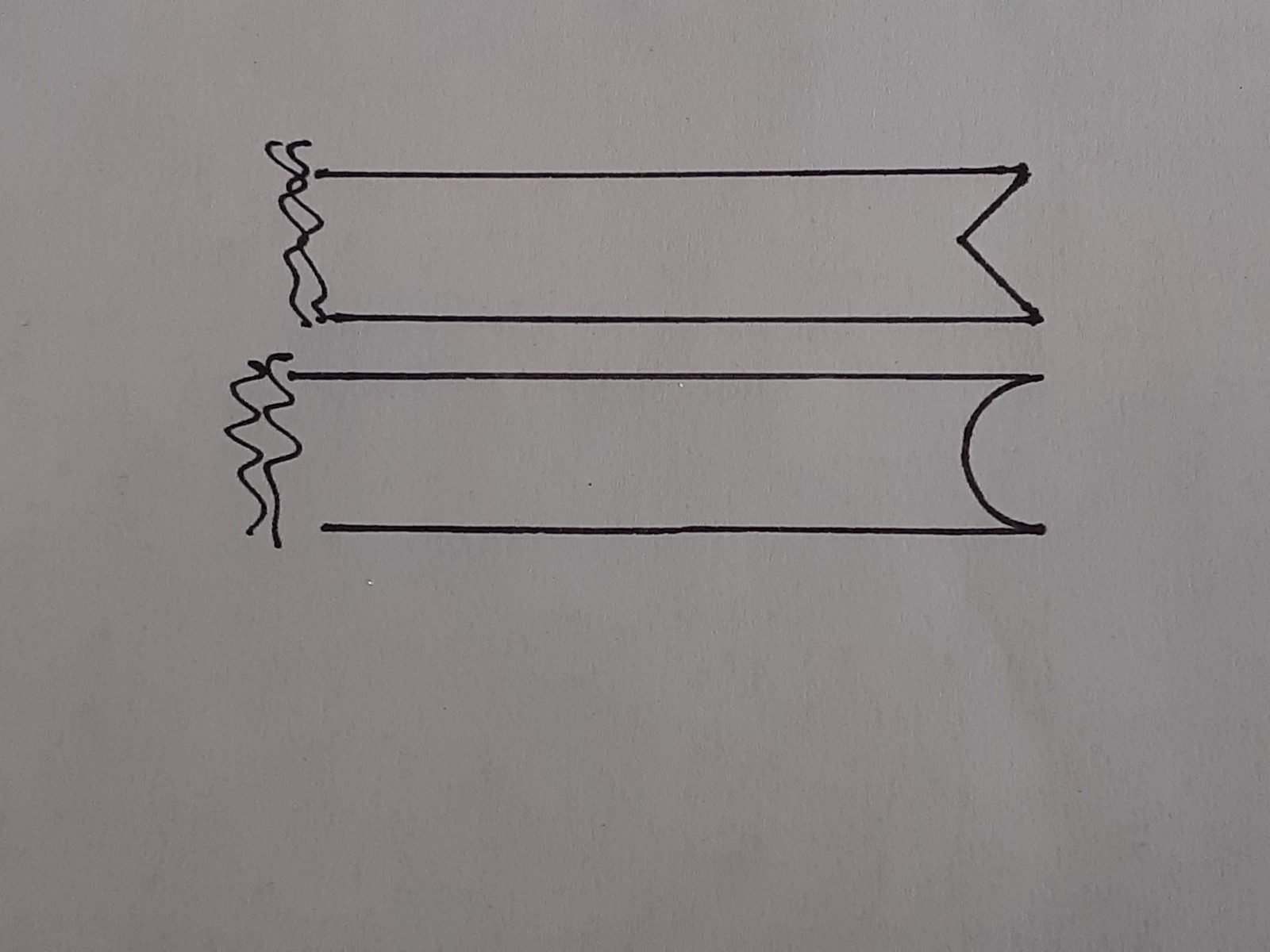In this image, we see a photograph featuring simple, dark black ink lines on a white sheet of paper, which appears light gray due to the low lighting conditions. The rectangular photograph has longer top and bottom sides compared to its left and right sides. In the top half of the image, two banner shapes are meticulously drawn. 

The left side of each banner features two squiggly lines, totaling four lines, with the top parts of these lines pointing towards the top edge of the photograph and the bottom parts pointing towards the lower edge. The upper banner takes on a rectangular form, complete with a triangular cutout on its right side. The banner directly below is also rectangular, but its right side is adorned with a semi-circular cutout, adding a gentle curvature to its design. The left edges of both banners remain open, devoid of any drawn lines.